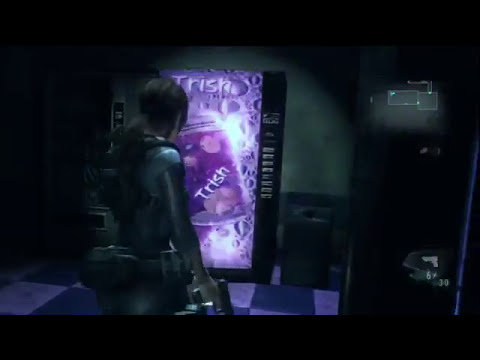A dimly lit hallway in a video game serves as the backdrop for this intriguing scene. Dominating the left-center is a character, identifiable as a woman by her ponytail, dressed in a dark, silverish-gray suit. Her outfit is equipped with a utility belt and a backpack, indicating she's prepared for action. She stands with her right hand gripping a sophisticated machine gun, partially visible, while her attention is fixed on a vending machine directly in front of her. 

The vending machine, adorned in various shades of purple, prominently displays the brand name "Trish" in light purple lighting at the top. A tilted soda can bearing the same name and surrounded by purple bubbles adds a touch of realism to the machine. The floor beneath the character features checkered black and white tiles, enhancing the overall dark ambiance.

In the game's interface, a mini-map located just below the top right corner indicates the player's location within the map. Meanwhile, the bottom right corner of the screen shows a pistol icon, symbolizing the selected weapon, accompanied by the numbers "6" and "30," denoting the rounds in the chamber and reserve ammo, respectively. The character is viewed from an over-the-shoulder perspective, capturing her from head to mid-torso.